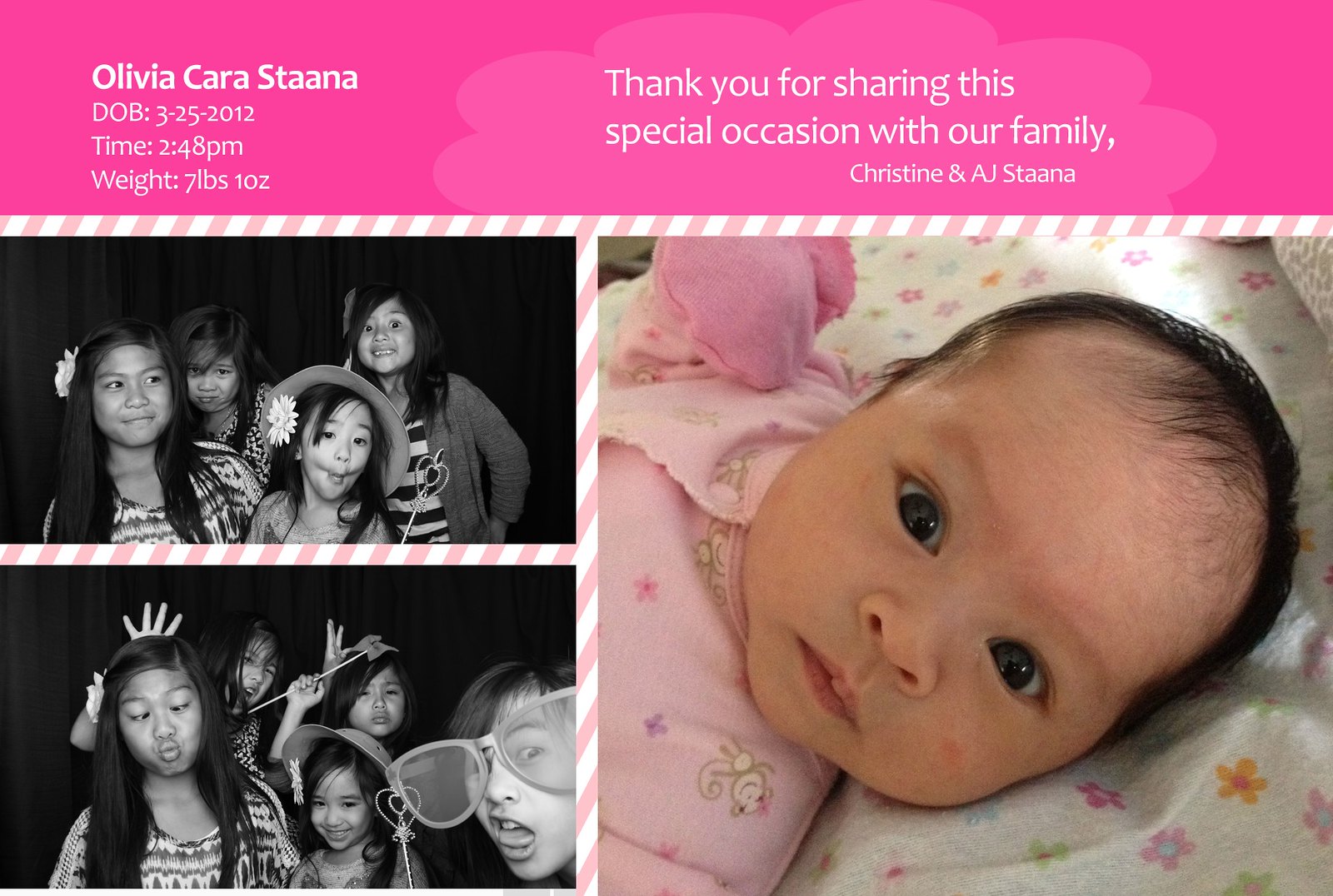This image showcases a horizontally aligned, rectangular thank-you card celebrating the birth of Olivia Cara Stana, born on 3-25-2012 at 2:48 p.m., weighing 7 pounds 1 ounce. The top section of the card features a bright pink banner with Olivia's name, birth date, time, and weight in bold, white letters on the left. Centered on this banner is a heartfelt message: "Thank you for sharing this special occasion with our family, Christine and AJ Stana." Below the banner, on the right-hand side, is a large, close-up photograph of a newborn baby girl with bright eyes, black hair, and wearing a pink dress featuring a monkey design and butterflies. To the left of the baby's photo are two smaller, horizontal black-and-white photos. The top shows four young girls making silly faces, while the bottom captures five girls, with one wearing oversized, goofy glasses, all posing playfully. These images likely depict Olivia's family members, adding a personal and joyful touch to the celebration of her birth.